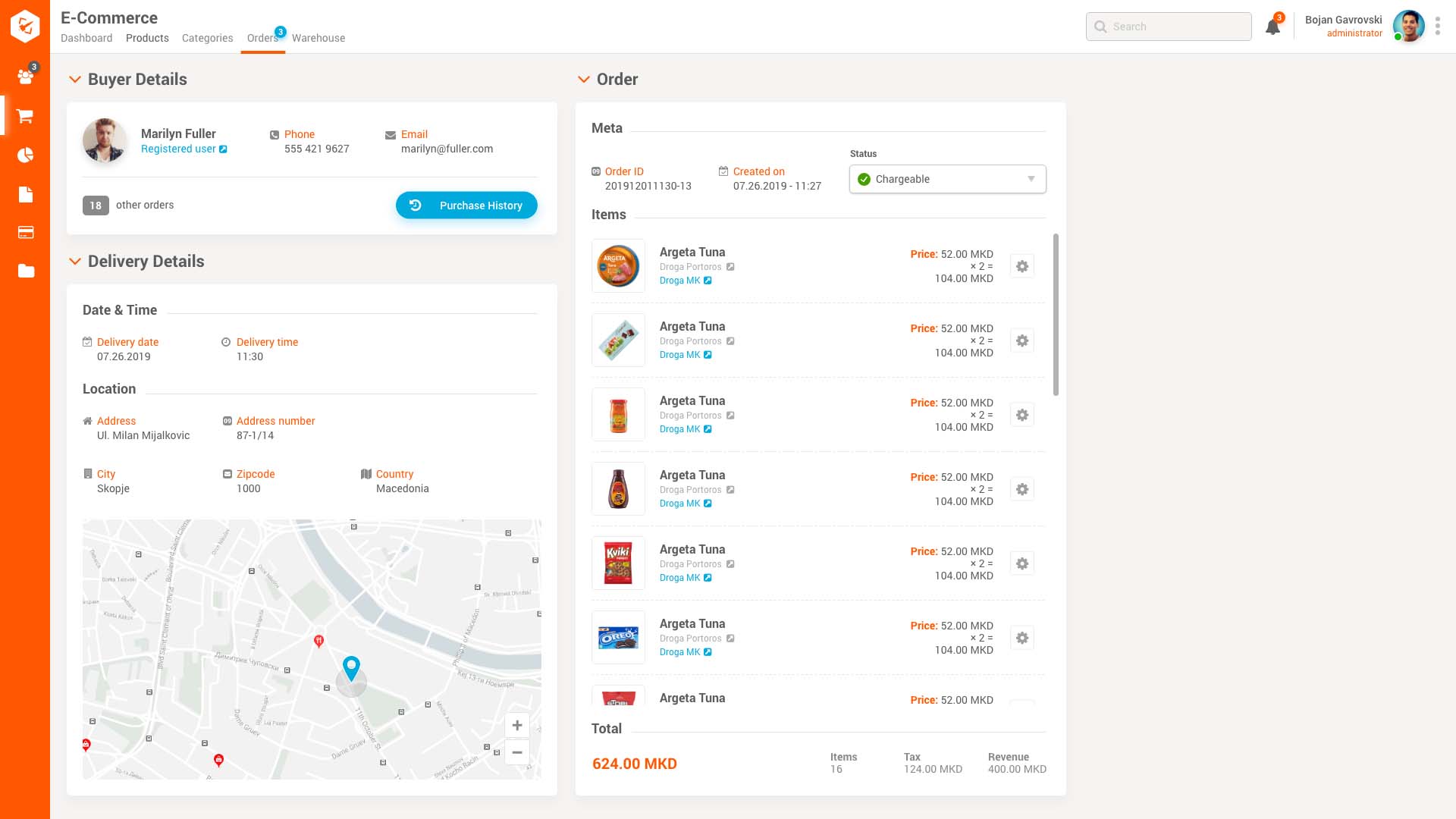The image depicts a detailed screenshot from an e-commerce website's dashboard. At the top of the dashboard, there are navigation labels: "Products," "Categories," "Orders," and "Warehouse," with the "Orders" section showing a notification of three new orders in a small teal circle.

Below the navigation, buyer details for a user named Marilyn Fuller, a registered user, are displayed. Contact information is shown with the words "Phone" and "Email" highlighted in orange, alongside the corresponding phone number and email address. A blue refresh button, which can be clicked to update purchase history, is present, showing that Marilyn Fuller has a total of 18 orders.

The left side of the image features a vertical, bright orange strip containing various icons, such as a paper document, a file folder, and a shopping cart, among others.

Towards the bottom of the image, the delivery details are outlined, including the date, time, and location of delivery, alongside a small map for reference. 

The order details section at the center of the image specifies a header labeled "meta" and includes the "Order ID" followed by a long numerical identifier. The creation date is marked as 07-26-2019 at 11:27 AM, with a checkmark indicating that the order is "chargeable." 

As you scroll down further within the image, the items in the user’s shopping cart are listed. The total amount for the order is displayed at the bottom, summing up to 624.00 MKD.